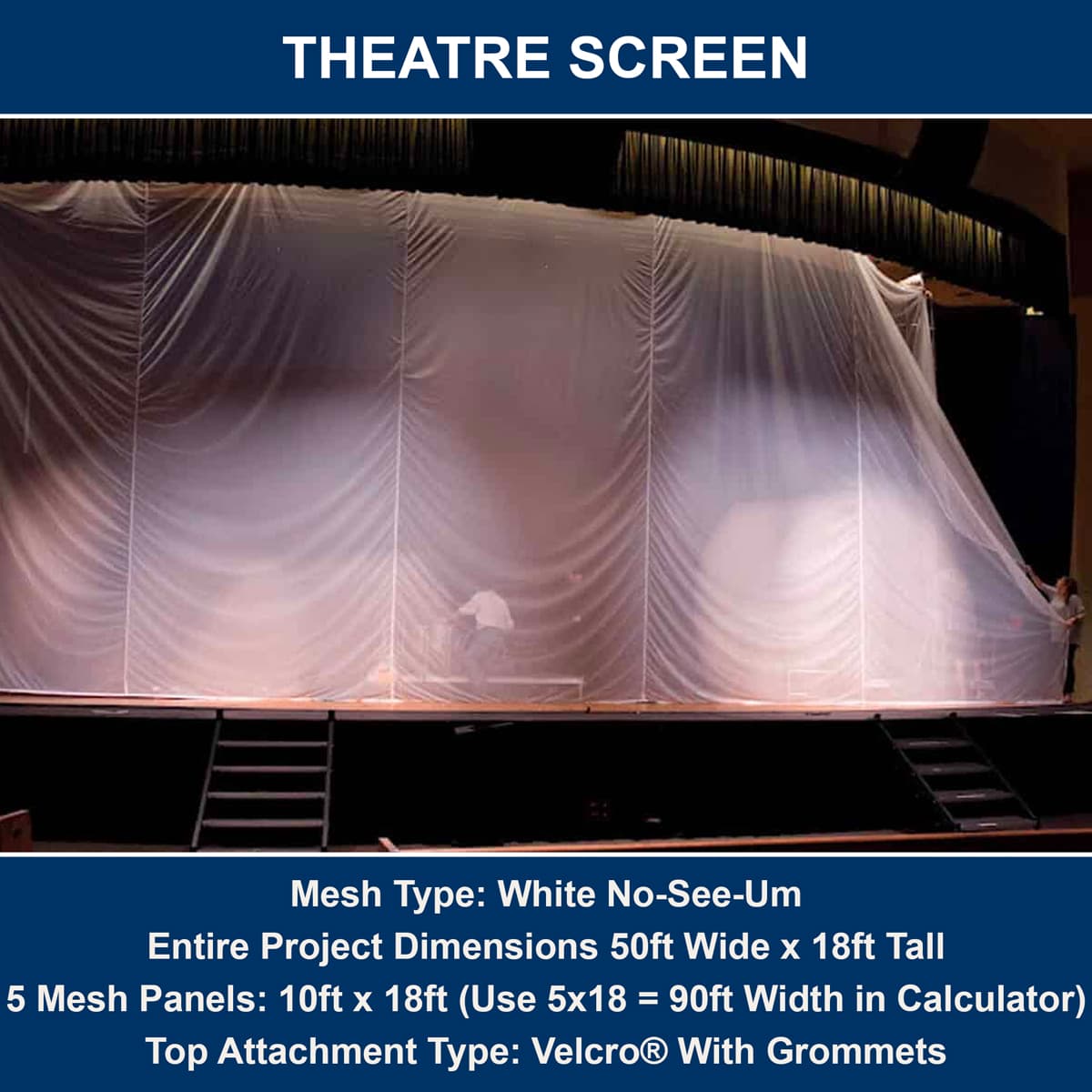The photograph showcases a theater screen labeled "THEATER SCREEN" at the top in white text against a blue background. The central image features a stage with a large, translucent screen made of white mesh panels sewn together. This screen, appearing almost like a curtain, hangs from a bar or sliding mechanism at the top and reaches down to the stage, creating a slightly rounded effect. The overall dimensions of the project are 50 feet wide by 18 feet tall, constructed from five mesh panels, each measuring 10 feet by 18 feet. Near the center of the screen, a person is faintly visible behind its semi-transparent fabric, adding to its see-through quality, while another person stands to the side of the screen, possibly adjusting it. Below the image, additional details are provided in white text on a blue background, specifying the mesh type as "white no-see-um" and noting that the top attachment utilizes Velcro with grommets.